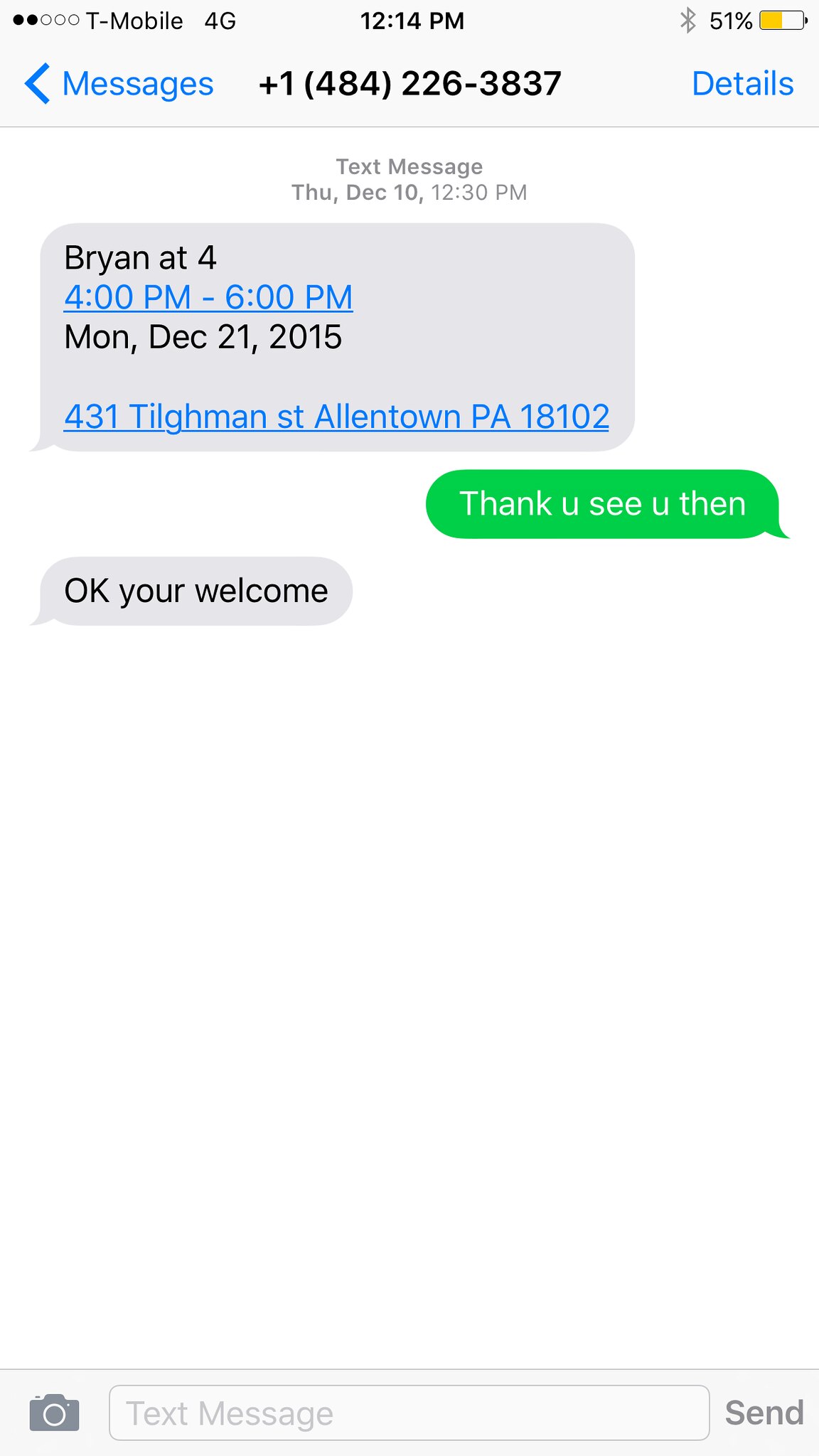The screenshot of a cell phone displays a text message conversation against a plain white background. At the top, the phone indicates it's on the T-Mobile 4G network with the time showing 12:14 PM, and the battery level is at 51%. The message is from the number 1-484-226-3837. The text message details are as follows: In a gray box, it states "Brian at four" in black text, followed by "4 PM to 6 PM" in blue text, and "Monday, December 21st, 2015" in black text. Below this, another blue text line provides the address "431 Tillman Street, Allentown, PA, 18102." The reply, displayed in green, states, "see, thank you, see you then," followed by a gray reply, "okay, you're welcome." The interface includes a text input box with a send and a camera button at the bottom.